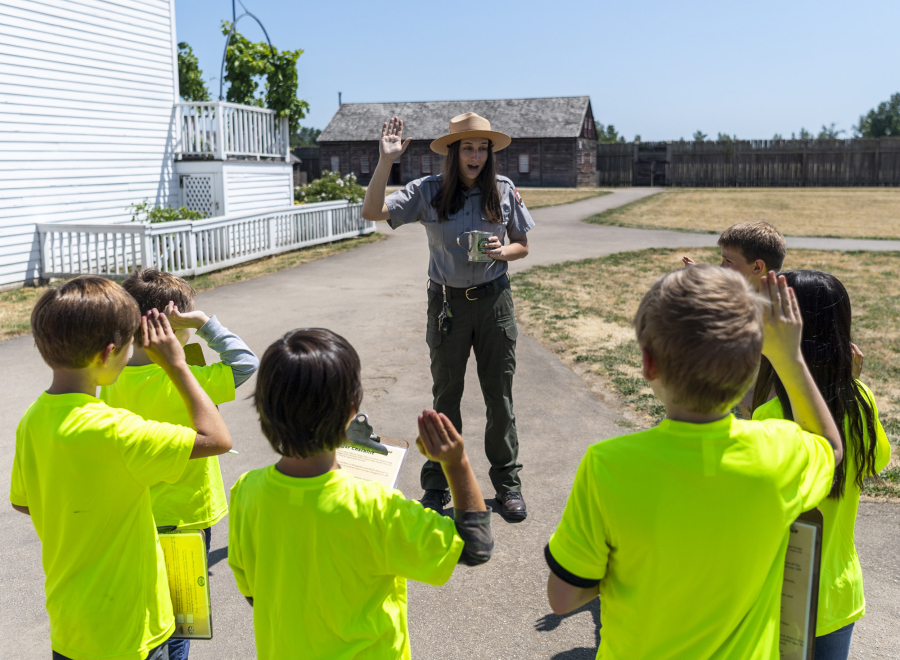In this engaging image, six children donning neon green shirts stand in a line with their right hands raised as if taking an oath. Each child clutches a clipboard in their left hand. From left to right, the first two children have short brown hair, the third has slightly longer black hair, and the fourth has short blonde hair. The fifth child is a girl with long black hair, while the sixth child’s features are less specified. Directly in front of them, a scoutmaster stands center stage, mirroring the children's raised right hand gesture. She holds a silver cup in her bent left arm. She is noticeable with her distinctive outfit, including a brown mounting hat, a short blue button-up shirt, green khakis, black boots, and a brown belt. Her long black hair flows over her shoulders. 

The backdrop reveals a rustic outdoor setting, with a wooden fence extending from the right towards the center, leading to a wooden building. Further left, a charming white house with a porch and white railings is partially visible. The scene is set on a roadway that meanders towards the fence in the distance, with another road diverging to the right halfway up. The bright, clear sky caps this delightful scene, suggesting a beautiful day filled with the joy of camaraderie and outdoor adventure.